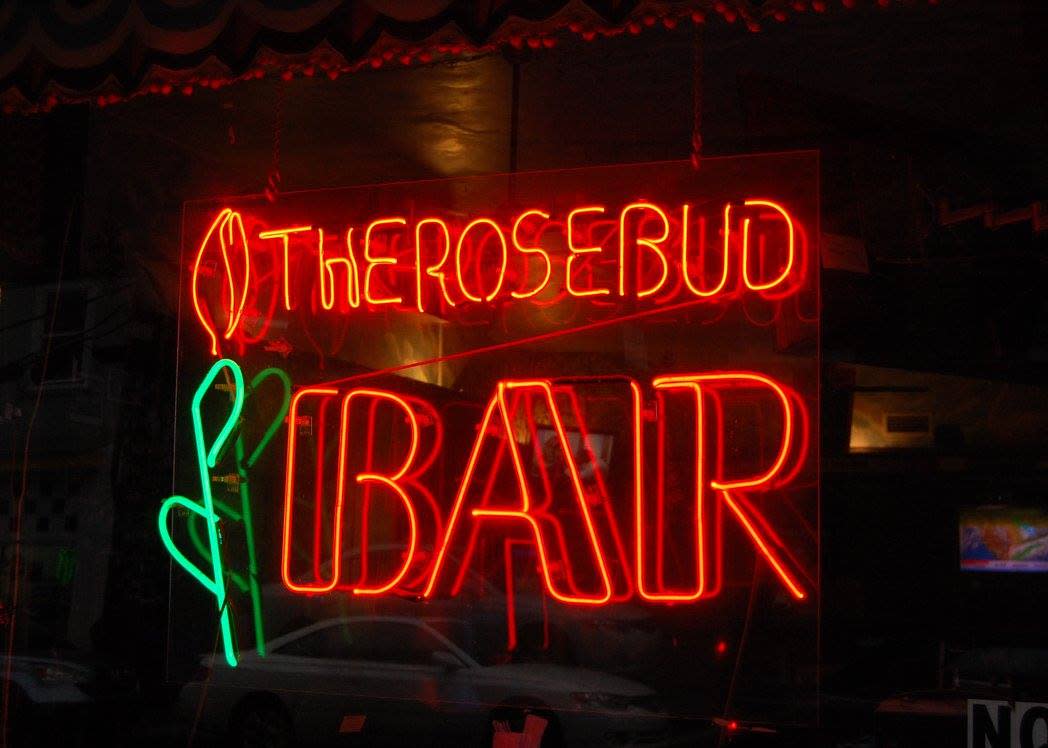This photograph captures a striking neon sign displayed in the window of a bar during nighttime, which enhances its vibrant glow. The red neon sign prominently features "BAR" in large, bold letters, situated beneath the smaller "The Rosebud" lettering at the top. Accompanying the text is a neon depiction of a rosebud with a red blossom and a green stem with two simple leaves, positioned to the left of the words. The dark surroundings make the neon colors stand out brilliantly, drawing attention to the establishment.

The reflections in the window add depth to the image. Visible are a white parked car and the inside of the bar, where a television is on, contributing to the cozy atmosphere. The photograph's setting is subtly adorned with some festive trim above the sign, hinting at a celebratory ambiance. The clarity of the neon sign against the clear, black background and the detailed reflections make this image captivating and reflective of its lively environment.